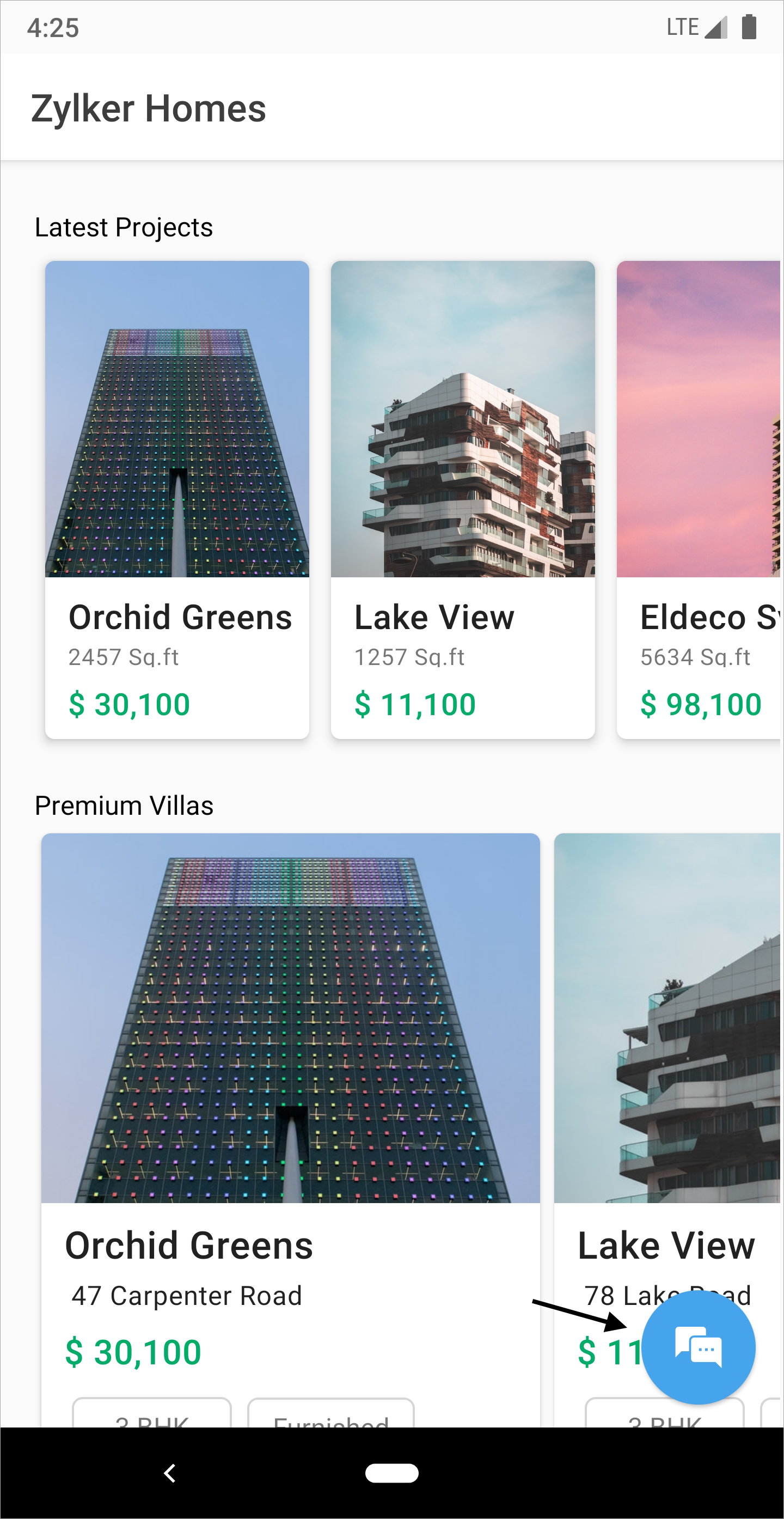At the top of the display, the screen shows '4:25' in the top-left corner and 'LTE' in the top-right corner. The service bar is nearly three-quarters full, and the battery icon is gray. Below that, 'Zilker Homes' is written in black on the left side. 

There is an option for "Latest Projects," displaying three options, although the third one is partially cut off. The first project showcases an image of a black skyscraper labeled "Orchid Greens," which is 2,457 square feet and priced at $30,100. The second project features a more contemporary skyscraper with a brick and white exterior, labeled "Lakeview," which is 1,257 square feet and priced at $11,100. The third visible project, set against pink skies, is labeled "ELDECO," which is 5,634 square feet and priced at $98,100. All price figures are highlighted in light green.

Beneath these options, there is a section labeled "Premium Villas," with "Orchid Greens" listed under this category. Three-quarters of the way down the page, there is an arrow pointing towards a blue chat bubble icon with white chat symbols inside it.

At the bottom of the page, a black bar contains a white 'V' pointing to the left, followed by a solid shape resembling a Tic-Tac in the center.